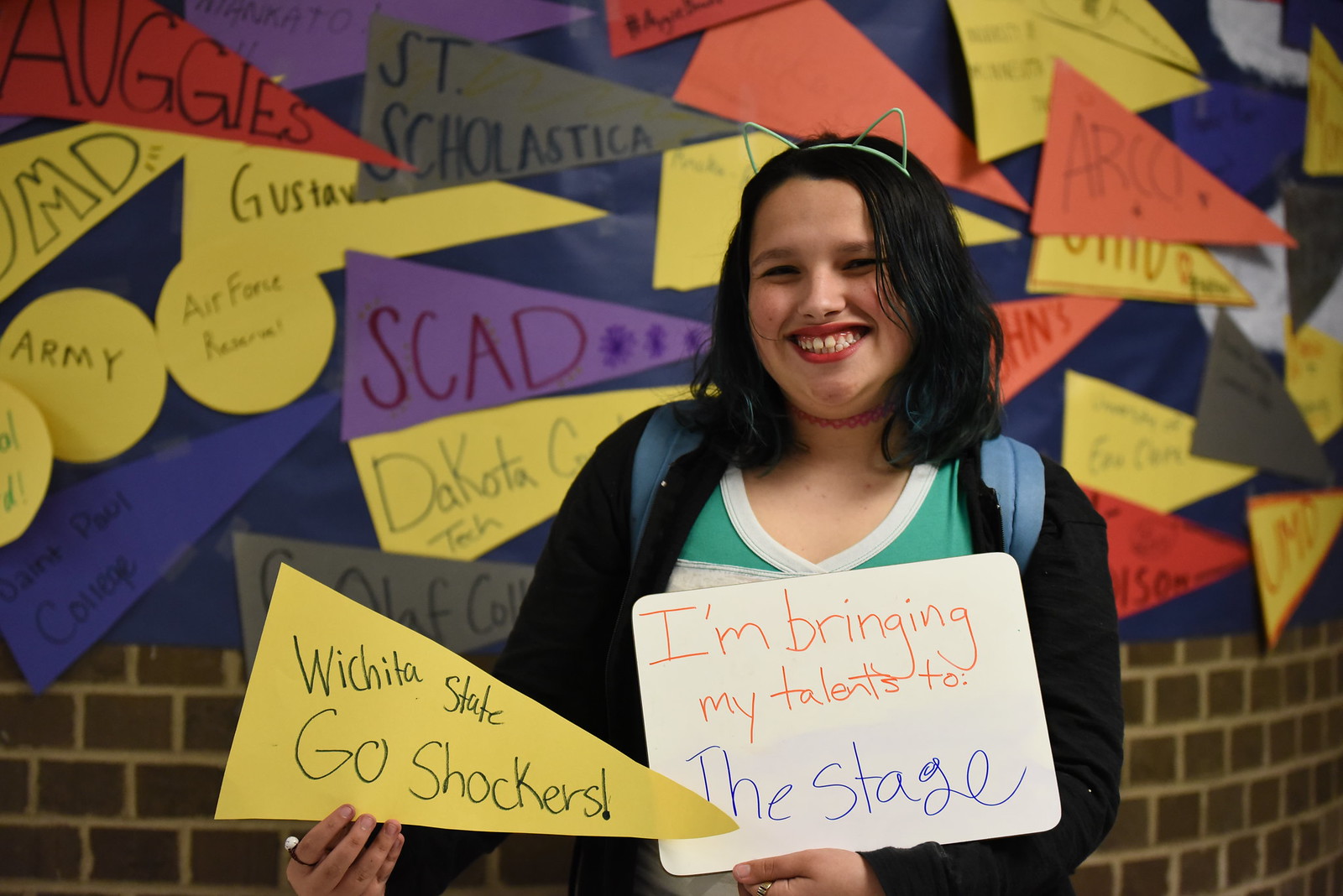The landscape-oriented color photograph captures a vibrant and joyful moment of a girl, approximately 14 years old, standing in front of a brick wall decorated with numerous colorful triangular flags, each adorned with various phrases. The girl is centered slightly to the right, beaming up at the camera with a wide smile, revealing her nice teeth. She is dressed in a black sweater over a blue and green v-neck shirt, and her shoulder-length black hair is complemented by a headband with white cat ears. On her back, she carries a blue backpack.

In her left hand, she holds a small whiteboard with handwritten text in red and blue markers that reads, "I'm bringing my talents to the stage." In her right hand, she proudly displays a yellow triangular pennant with the inscription "Wichita State Go Shockers" written in black marker. The background's brick wall is painted in shades of algae green and yellow and is adorned with a variety of colorful paper pennants, featuring words like "Saint," "Scholastic," "SCAD," "Dakota," "Army," "Aviation," and "Air Force." The photograph is a delightful and detailed representation of youthful exuberance and school spirit, set against a vivid and eclectic backdrop.